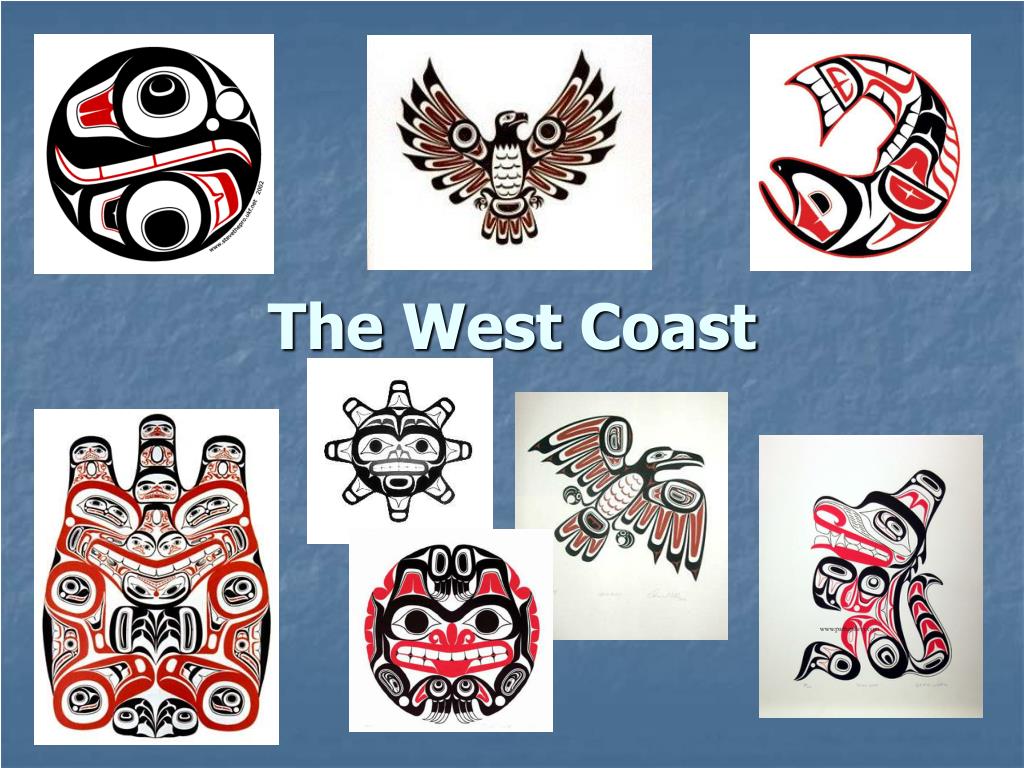A detailed display on a blue background showcases a central white text reading "The West Coast," surrounded by eight culturally-rich images reflecting Northwest Indian totems, each rendered in black, red, and white. Starting at the top left, a round decoration features intricate black and red designs. Adjacent to it, an eagle or phoenix with outstretched wings contrasts boldly against the background. To its right, a stylized fish, curved with an open mouth, adds dynamic flair to the composition. The lower left corner holds a group of dolls enshrined in tribal artistry. Near it, series of facial images include a sun-like design radiating with thick black and white spokes. Following this, a tribal mask face is encased within a circlet and a stylized bird, reminiscent of a pelican, is depicted in flight. The final image to the far right intricately presents a face belonging to a serpent, distinguishable by a hat, weaving an aura of mystique. The collection seamlessly intertwines visual storytelling with tradition, encapsulating the essence of the West Coast's indigenous heritage.